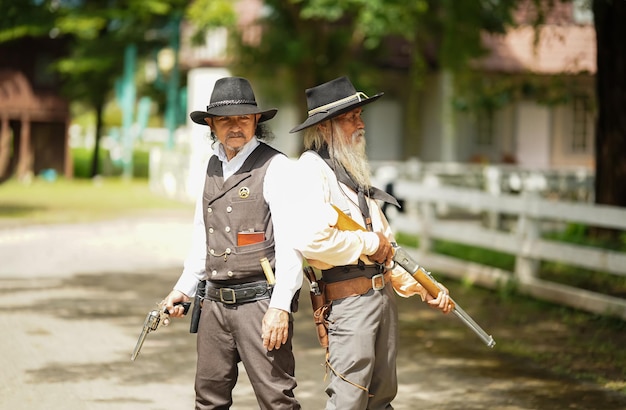In this image, two men stand back-to-back, their shoulders touching, in what appears to be a recreation of an old Western scene. Both men are wearing white shirts and black cowboy hats. The man on the left is dressed in a gray vest with a sheriff's star, gray pants, and a black belt. He holds a silver pistol in his right hand, and a holster with another gun is visible on his waist. His outfit also includes a black half-jacket with five buttons arranged in rows of two and a bottle tucked into one of its pockets. The man on the right, sporting a gray beard, is equipped with a long brown and black rifle. He's also wearing a white shirt, gray pants, and a black bandana around his neck, with a brown belt and a gun holster at his waist. A picket fence, houses, and green vegetation are all visible in the background, indicating that the photo was taken on a sunny day. The detailed scene suggests a staged, modern interpretation of the Old West, complete with thematic costumes and props.